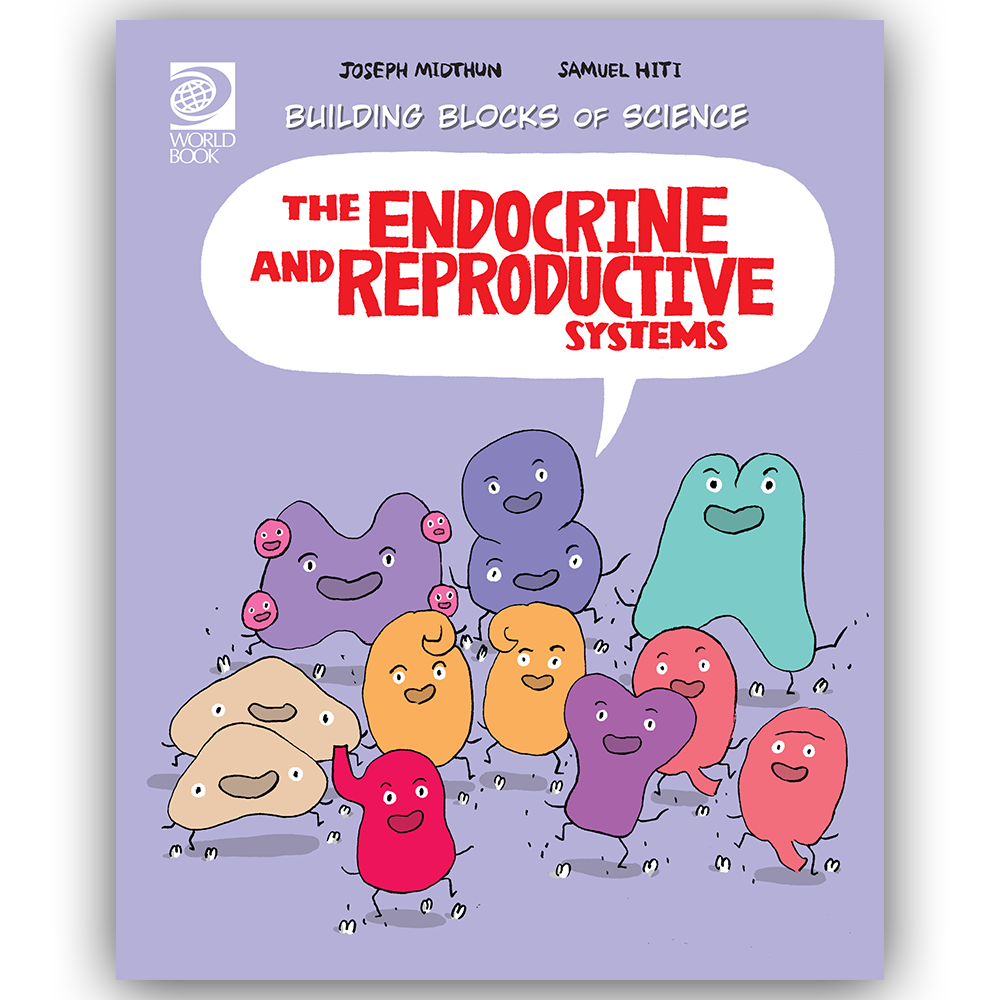This image depicts the cover of a children's book titled "Building Blocks of Science: The Endocrine and Reproductive Systems," authored by Joseph Midthun and Samuel Hiti and published by World Book, whose logo appears in the top left corner. The cover features colorful and simplistic depictions of various organs from the endocrine and reproductive systems designed in a playful, child-friendly manner. These animated organs, including representations of testicles, a vagina, ovaries, and a sweat gland, are illustrated as smiling, dancing blobs in various colors such as purple, yellow, red, tan, pink, and green. The background of the cover is a light purple, creating a lively and engaging visual meant to educate children in an accessible way.